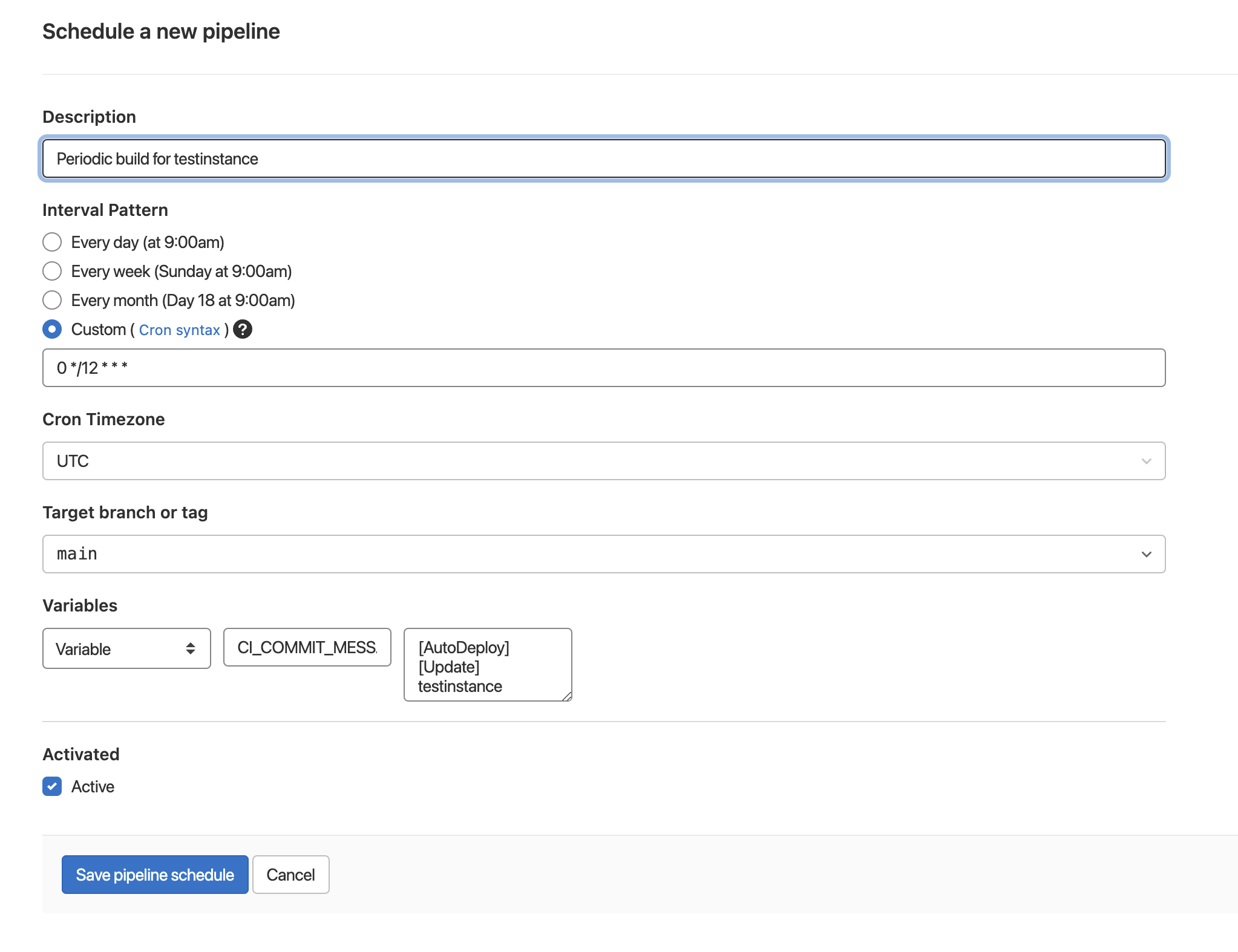The image depicts a section of an online form, likely related to scheduling a pipeline. The form has a mostly white background with black text. 

At the top, there is a black header that reads "Schedule a New Pipeline," followed by a thin horizontal grey line. Below this, the form contains sections such as "Description," with a bordered box highlighted in black and blue. The description box reads "Periodic build for test distance."

The form segment includes definitions under "Interval Pattern," displaying several options in red-bordered boxes:

1. Every day at 9:00 AM
2. Every week on Sunday at 9:00 AM
3. Every month on the 16th day at 9:05 AM
4. Custom option, which is selected (checked).

Within the custom option, there are fields for inputting custom scheduling parameters, described as symbols and containing fields like "0/112."

Additional fields are visible:
- "Cron Time Zone: UTC"
- "Target Branch or Tag: main"
- A variable field labeled "CCCMTMESS."

Another section contains an "Auto Display Update" box labeled "Test Disturbance Activated" and an "Activate" checkbox which is checked, indicating this feature is active.

At the bottom, a light grey band spans the form with two blue buttons labeled "Save Pipeline Schedule" and a white "Cancel" button.

This detailed structure suggests it is a configuration interface possibly for setting up automated tasks or maintenance schedules within a software pipeline, although the exact purpose is somewhat ambiguous.